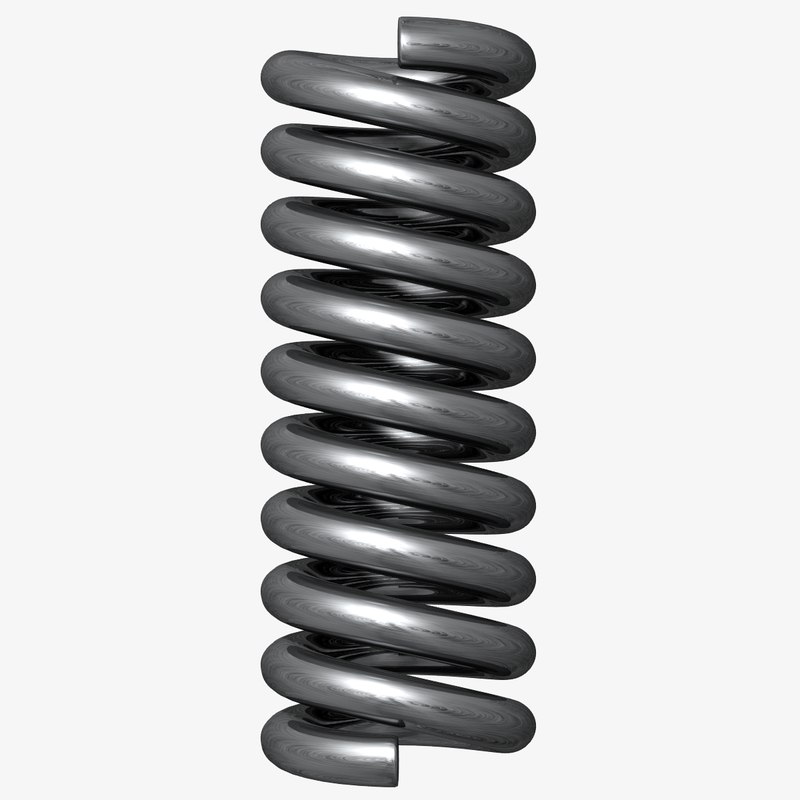This detailed illustration captures a vertically positioned, metallic coiled spring, likely resembling a shock absorber, against a clean, white or eggshell background. The shiny, dark silver metal coils uniformly wrap around approximately ten times, creating a thick and potentially very springy structure. The spring's intricate shading and uniform design suggest it might be an illustration rather than a photograph. The minimalistic composition enhances the focus on the spring itself, highlighting its well-defined, evenly spaced coils and the ends visibly tapering at the top and bottom.